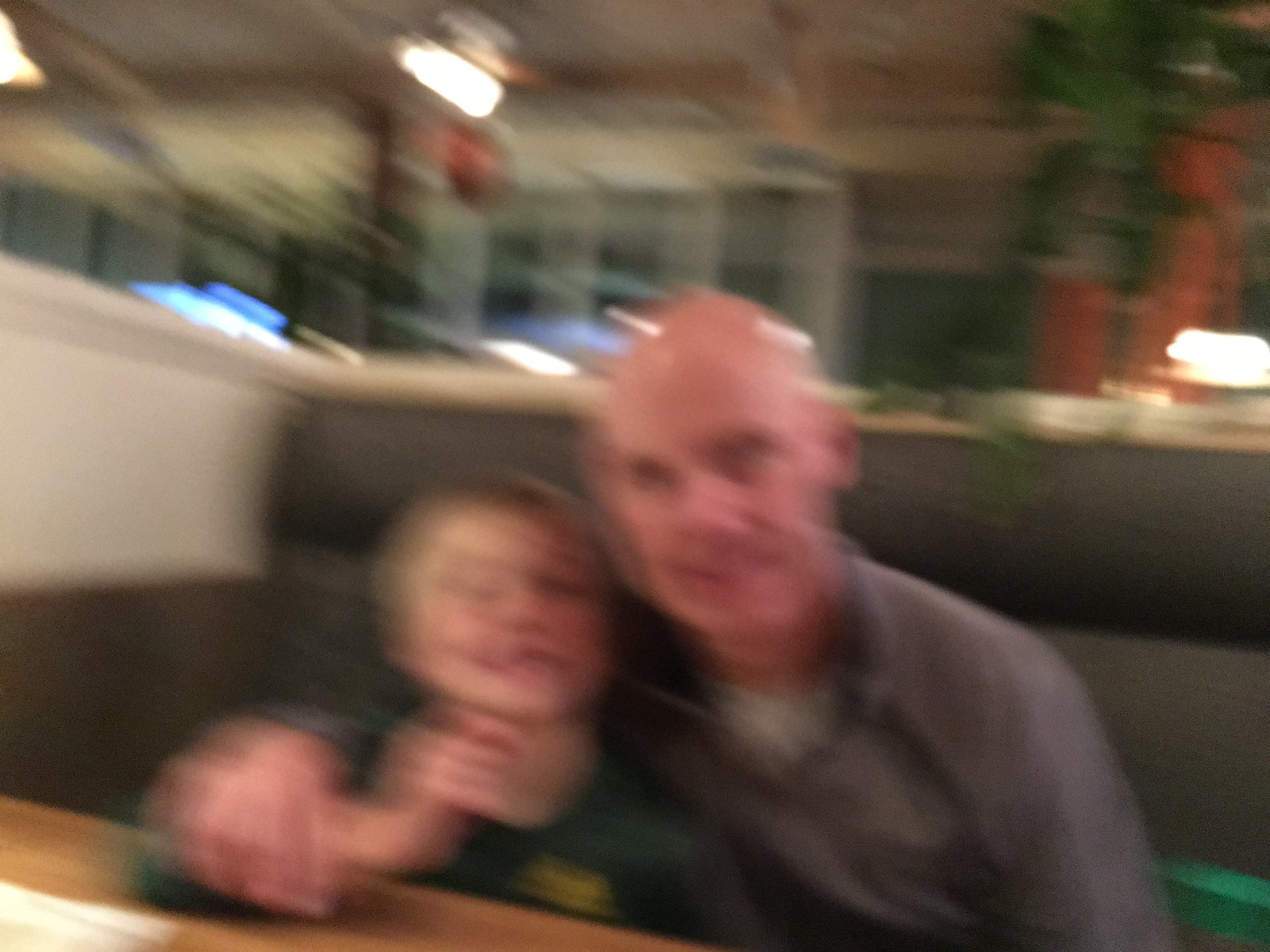In this notably blurry photograph, a man and a child are seated together in what appears to be a restaurant booth. The man, bald and wearing a dark grey shirt with a white undershirt, has his right arm wrapped around the child's shoulders. The child, who has brown hair and is dressed in a green shirt featuring yellow writing on the right side, sits to the man's left. Both are smiling and looking directly at the camera. The booth they occupy has dark padding that extends above their shoulders, and a golden brown wooden table is positioned in front of them. The background includes a wall and windows with white borders and some brown elements, as well as reddish-pink pillars. The overall image quality is very poor, with significant blurriness and signs of motion during capture, giving the scene a somewhat out-of-focus appearance.